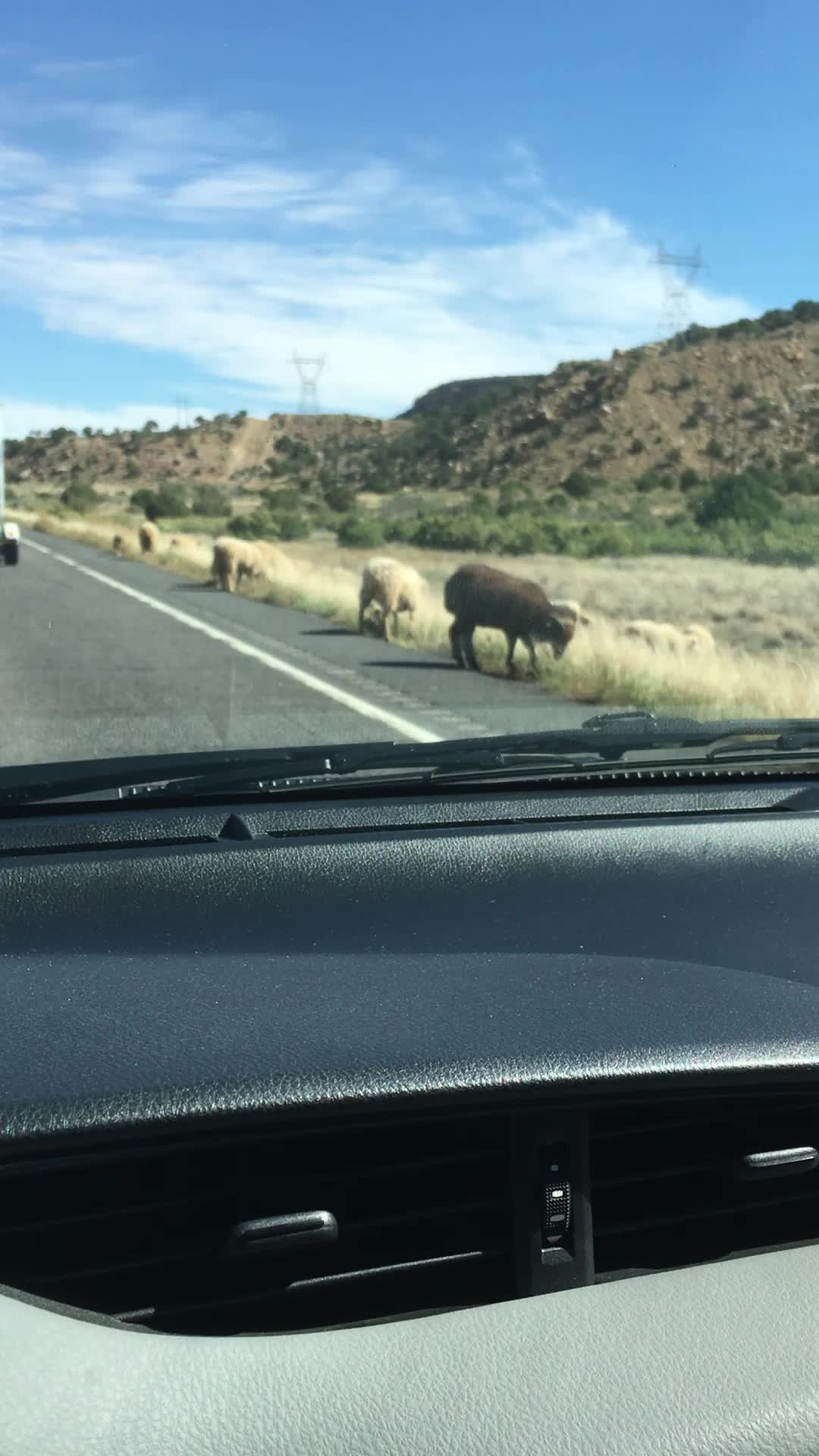The image captures a scene from inside a car, looking outward through the windshield. Central to the scene, four sheep are grazing on the edge of a road, their heads lowered to a light yellow grassy field. Among them, one sheep stands out with its dark brown coloration, while the other three are lighter in color. The backdrop features brown hills and mountains, adding depth to the landscape. In the distant background, several towers, possibly cell phone or electrical, rise above the horizon. The foreground of the image includes the car's black dashboard, visible air conditioner vents, and the black windshield wiper positioned outside.